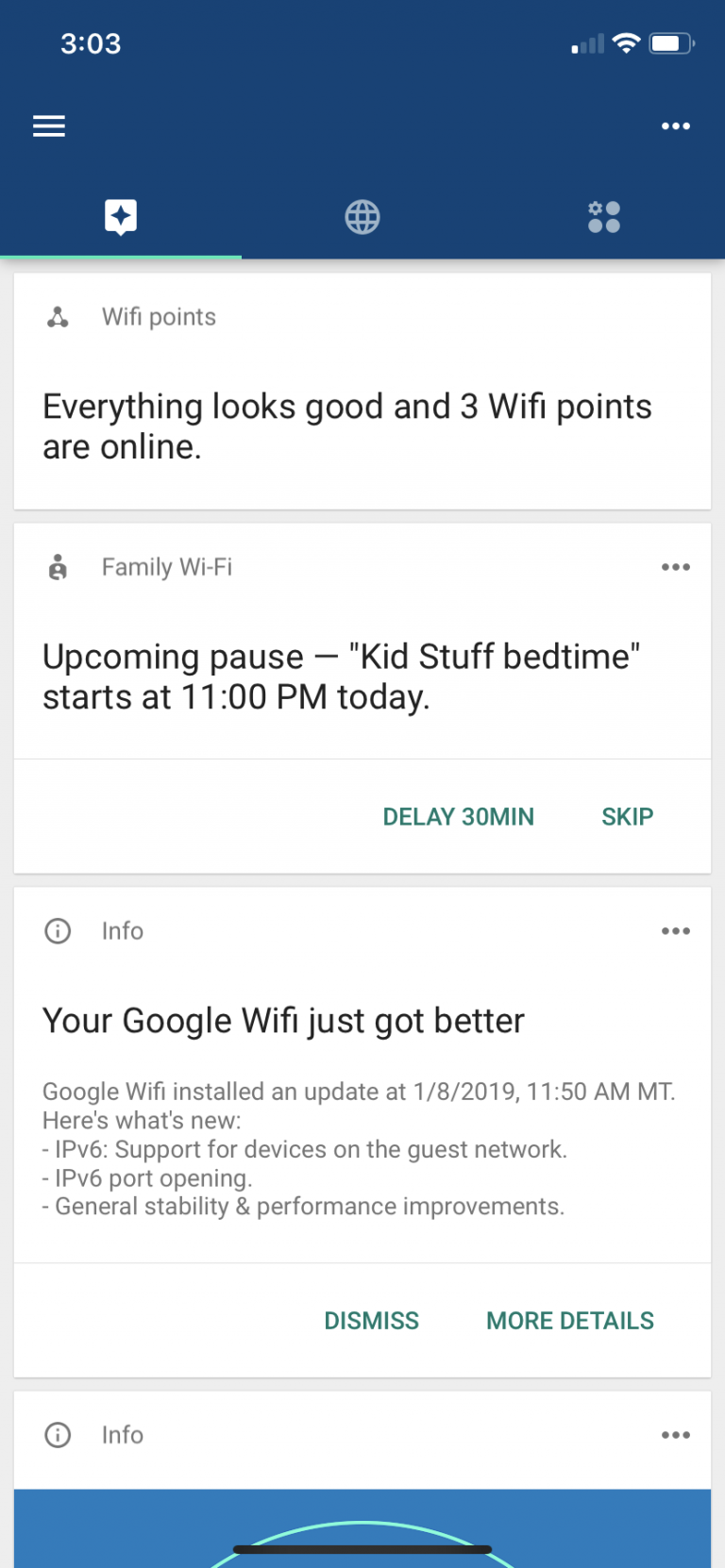A screenshot from a mobile device displays a user interface with detailed information and settings. At the top of the screen, there is a thick blue bar. Inside this bar towards the top left corner, the time "3:03" is shown in white text. Next to the time, there's a menu icon also in white. The status indicators show a cell signal with only one out of four bars, a fully maxed-out Wi-Fi signal, and a battery level of approximately 75%.

Below the blue bar, there are three tabs: one with a square containing a star, one with a globe symbol, and one with three white dots arranged in a vertical line, accompanied by a settings icon in the top left part of this section.

Further down, the screen displays Wi-Fi status with a message reading "Wi-Fi points: everything looks good" and indicating that three Wi-Fi points are online. 

Below this section, there are settings for Family Wi-Fi, detailing an upcoming pause for "Kids Stuff," which initiates a bedtime schedule starting at 11 p.m. today. Options to delay this pause by 30 minutes or skip it entirely are available.

Further down, there is information regarding updates, noting that "Your Google Wi-Fi just got better." The update was installed on January 8, 2019, at 11:50 a.m. Mountain Time. The update includes new features like IPv6 support for devices on the guest network, IPv6 port opening, and various stability and performance improvements. Two buttons are available at the bottom: one to "See More Details" and another to "Dismiss" this information.